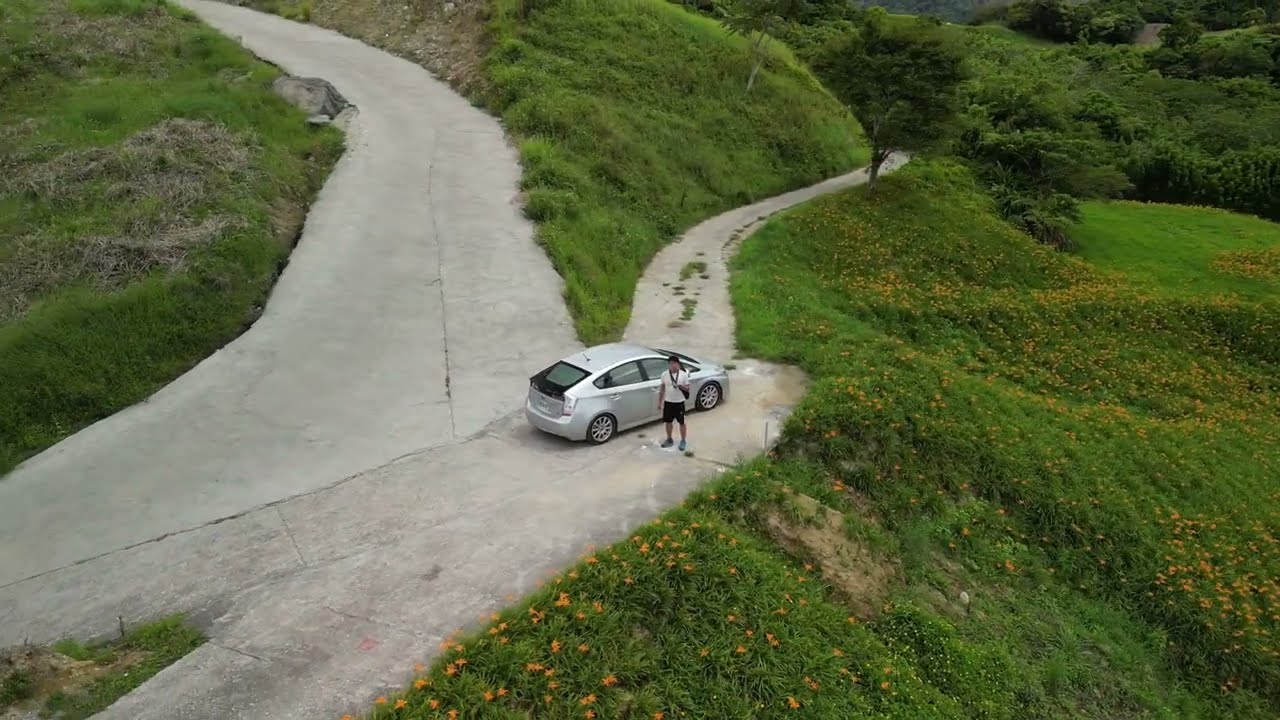In this vivid rural scene, a silver hatchback car is park on a narrow, concrete-paved roadway, which splits into two paths. One path curves smoothly up the hillside to the left, featuring a noticeable crack down the middle. The other path is much narrower, almost resembling a driveway, with grass growing in its center. Standing beside the car is a person in black shorts and a white t-shirt, who appears to be contemplating which path to take. This individual has dark hair and is striking a pose with one hand at his hip and the other near his chest, possibly looking towards the camera. The hillside surrounding the road is lush with billowy green grass, some of which is adorned with yellow and orange flowers. In the distance, on the upper right, a dense collection of leafy green trees adds to the natural beauty and seclusion of the area.